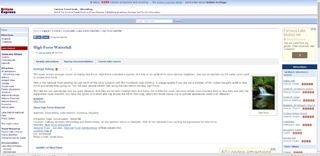This image depicts an outdated, low-resolution web page, likely from the early 2000s or late 1990s. The page has a primarily white background with black text, interspersed with some red and blue text elements. A notable feature of the page is an image of a waterfall, accompanied by text that appears to describe or name the waterfall, although it’s challenging to read due to the low resolution. 

At the top of the page, slightly towards the left, there's a search box. The left side features a column with various sections listed down its length, while the right side contains another column with red squares that could be ratings or some other form of indicators. The overall design is simplistic and reminiscent of web layouts from the Windows 97 or XP era, highlighting its age and lack of modern updates.